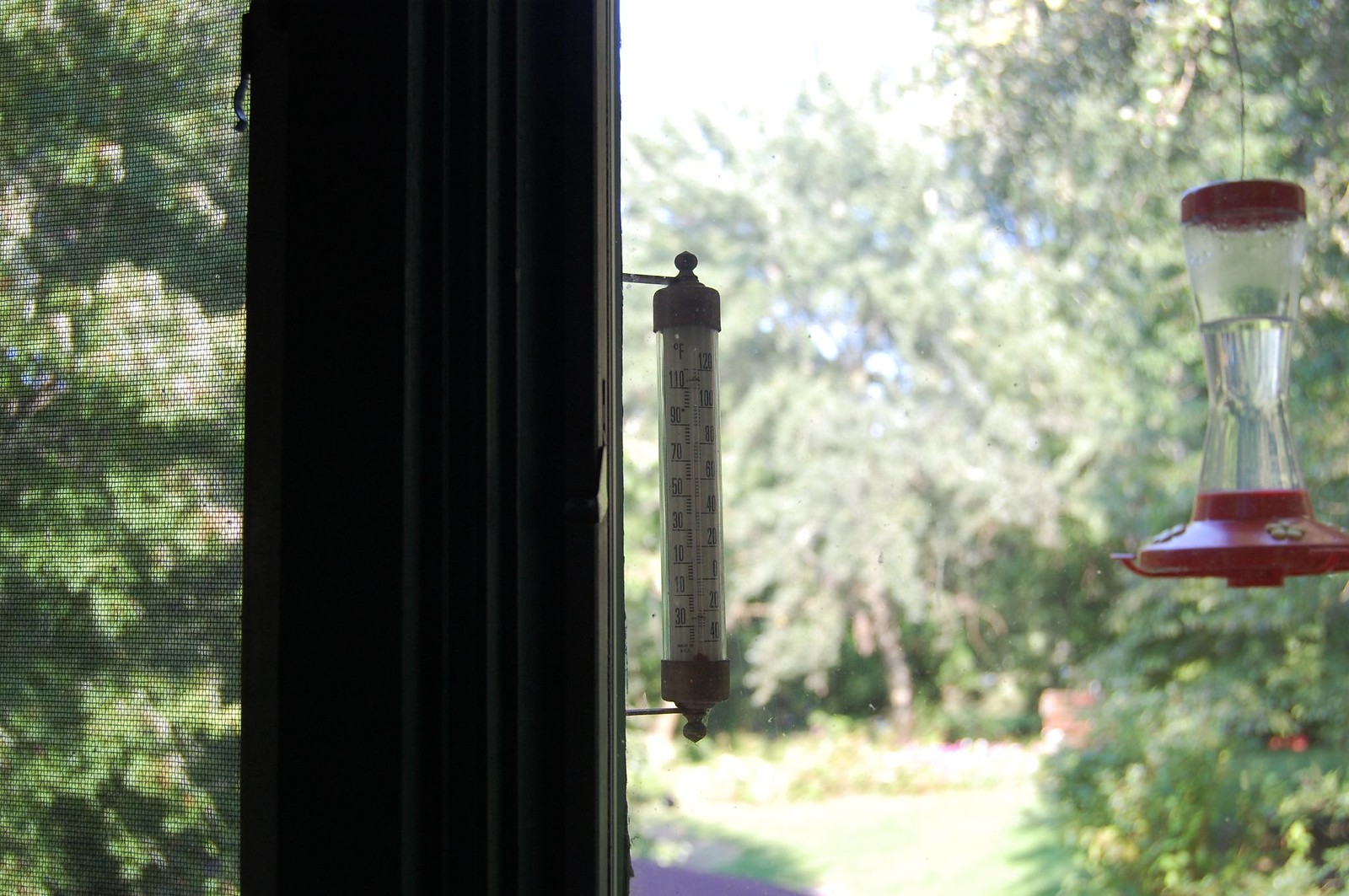The image showcases a detailed view of a temperature reader mounted on a wooden frame. To its left, an interesting object hangs from a string. The object is cylindrical with transparent sides, a red top, and a red bottom, and contains water filled halfway up. The temperature reader, prominently displayed next to the hanging object, has dual scales: one side displays temperatures in Fahrenheit, ranging from 30 to 110 degrees, while the other side shows a more detailed scale with markings at intervals of 20 degrees from 0 to 120 degrees.

In the background, a screen is visible, allowing a glimpse of the lush greenery outside. To the left, a variety of trees and bushes flourish, covered in vibrant green leaves and bathing in the warm sunlight. The sun illuminates the scene, casting light onto the grass and enhancing the vividness of the natural scenery outside.